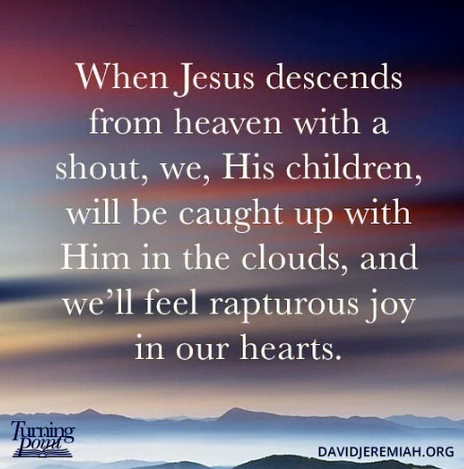The image portrays a vivid sky transitioning through various intense colors—shades of red, blue, purple, white, yellow, and pink—that create a captivating backdrop. At the bottom of the image, the horizon is lined with distant mountaintops rendered in bluish-gray tones. Central to the scene is a meaningful religious quote in bold white letters, stating, "When Jesus descends from heaven with a shout, we, his children, will be caught up with him in the clouds and will feel rapturous joy in our hearts." In the bottom left corner, the word "Turning Point" is featured alongside an image of an open book, while the bottom right corner reads "davidjeremiah.org."